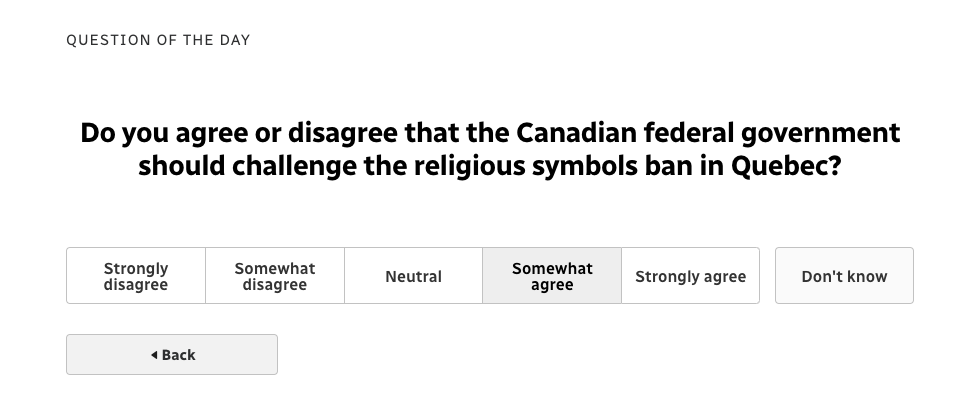The image features a clean, white background with the header "Question of the Day" prominently displayed at the top in large, bold black letters. The central question posed is: "Do you agree or disagree that the Canadian federal government should challenge the religious symbols ban in Quebec?" Below the question, multiple response options are presented in individual boxes: "Strongly Disagree," "Somewhat Disagree," "Neutral," "Somewhat Agree," "Strongly Agree," and "Don't Know." Notably, the "Somewhat Agree" option is highlighted in purple, indicating it has been selected. Additionally, a purple "Back" button is situated at the bottom, allowing users to navigate to the previous page.